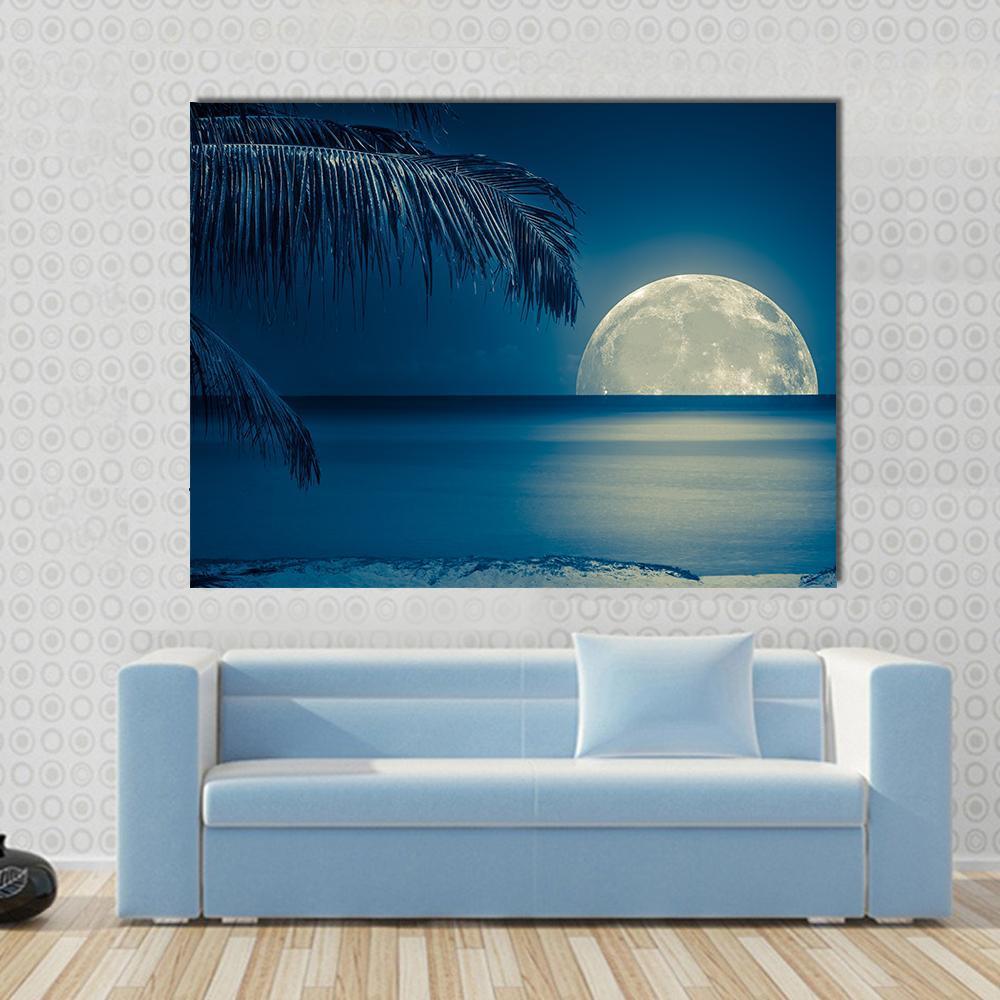In the artist's rendering of a serene living room, a light-colored hardwood floor stretches across the space, hosting a modern, light blue couch adorned with a single rectangular blue pillow on its right side. Dominating the wall above the couch is a large, captivating painting. This art piece depicts a tranquil night scene with a crescent moon illuminating a vast, blue ocean. The moon, positioned on the right-hand side, casts its reflection across the water, creating a dreamlike vista that includes palm trees gently intruding from the left and a slender strip of sandy beach in the foreground. The wall itself features an intriguing design of circular patterns in shades of white and gray, further enhancing the sophisticated ambiance of the room. A small black object rests discreetly on the left side of the couch, adding a subtle touch of contrast to the overall composition.